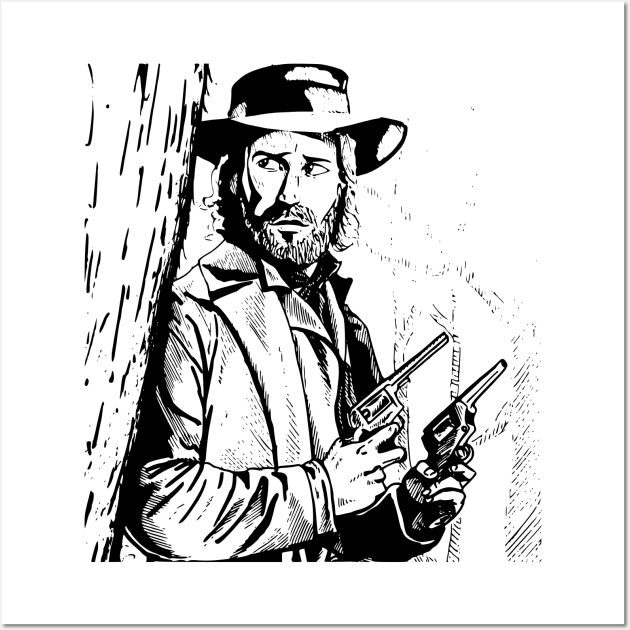This black and white image is a detailed pen-and-ink or pencil drawing resembling a panel from a cartoon strip. Central to the composition is a rugged cowboy, depicted with a black leather-look cowboy hat, a wide lapel jacket over a vest, and a knotted kerchief around his neck. His facial features include a beard and long hair that falls to his chin, and his eyes are shifted towards the left, peering cautiously around the tree as if on high alert for an approaching threat. The cowboy is holding classic 1800s-style revolvers in each hand, pointed towards the right side of the image, with the guns cocked and ready to fire. The tree trunk he leans against dominates the left side of the drawing, intricately detailed with bark texture. The background is sparse, with minimalist sketches of tree branches, indicating a forested area. Overall, this line drawing, rich in texture and shading, conveys a tense, high-stakes scenario in a Western setting.